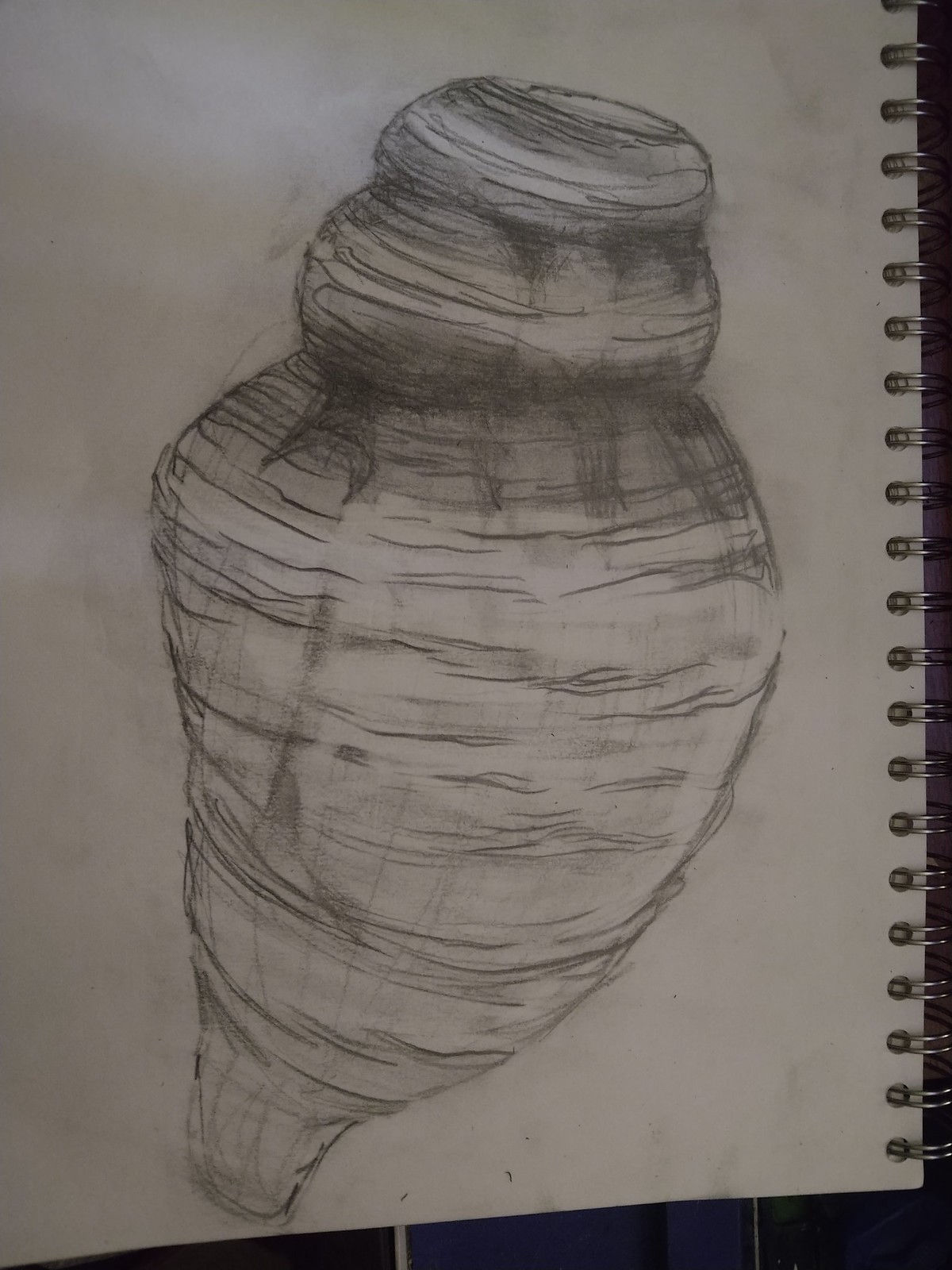The image showcases a meticulously arranged scene featuring various objects. On the right-hand side of the composition, there is a spiral-bound notebook, offering a subtle yet structured detail with its lined white paper casting gentle shadows. In the center foreground, an intriguing white object, possibly a shell or a vase, captures attention with its distinctive form. At its top, dark shadings interplay with segments of black and white, giving it a textured, almost three-dimensional quality. The shell's midsection is adorned with a triangle and encircled by intricate dark shadowing and numerous lines that add a sense of complexity and depth. To the bottom left of the image, there appears to be a hint of blood, rendered starkly in black and white, adding an element of contrast and possible intrigue. Tiny shavings are also visible near the bottom, suggesting recent erasing activity. The backdrop consists of uneven black tile, providing a textured surface that further enhances the overall aesthetic with its minimalist approach.